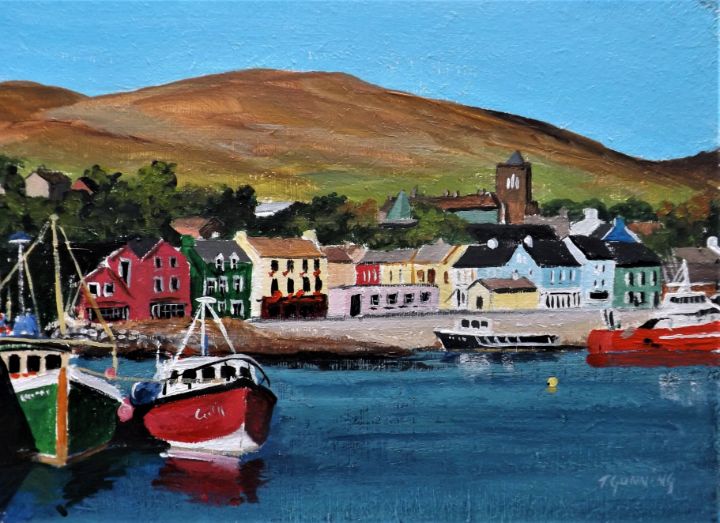This is a painting, likely an impressionist piece, either done in oil or watercolor, depicting a serene marina in a quaint village. The clear, bright blue sky crowns the scene, with brown hills and a row of green trees in the distance. Below the hills, a charming waterfront village is populated with a variety of 19th-century style buildings, including row houses and possible commercial buildings. These structures showcase a palette of colors: red, green, yellow, pale blue, and beige.

In front of the village, a busy dock extends into the blue water of the harbor. The harbor hosts several brightly colored boats; notable are two red and white boats, alongside a green and white one. Reflections and shadows of these boats ripple in the water, adding depth to the scene. Near the docks, there’s a small yellow buoy floating on the surface. The foreground is detailed with the water meeting a strip of dirt land, where the artist’s signature is subtly inscribed in a light shade of blue, blending harmoniously with the water.